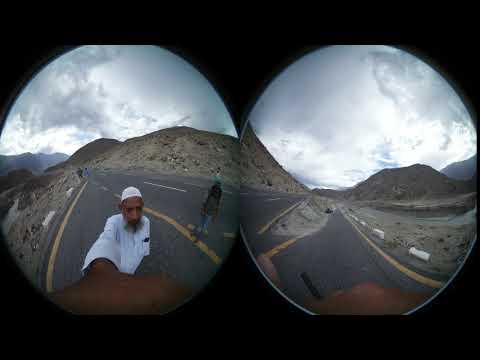The image is a digital photograph taken through two round lenses, portraying a man taking a selfie on an empty road. The left lens captures the man wearing a white shirt and white cap, holding up a camera with a selfie stick. Behind him, an empty black pavement road lined with yellow and white lines stretches into the background, flanked by white blocks. The sky is heavily covered with clouds, and in the distance, hilly, rocky, mountainous terrain devoid of vegetation is visible. Additionally, there is another man to the left of the main subject, dressed in blue jeans, a black and brown coat, possibly walking on this side road that veers off from a main road. The right lens of the image emphasizes the open roadway and landscape, including part of the man's hand holding the camera, but no other people or significant objects are in view. The color palette primarily features yellow, gray, brown, dark green, white, and blue.